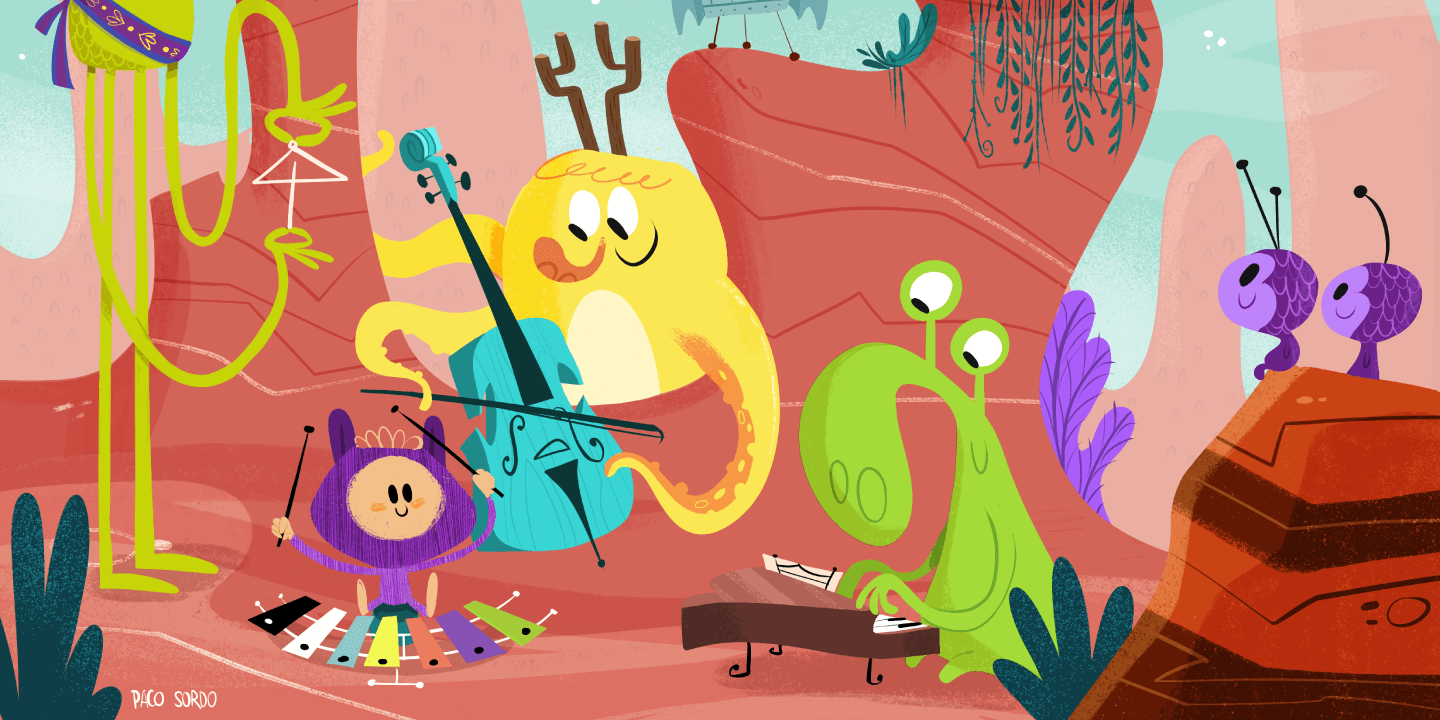The image portrays a vibrant and whimsical cartoon artwork set in a desolate, desert-like landscape dominated by red and pink cliffs with green vines dangling from them. The background features swirling, teal hues that add to the fantastical setting. Central to the scene are six cheerful, non-threatening monster characters, each vividly colored with exaggerated features. Among them, a lanky green figure adorned with a purple headband and elongated limbs plays a triangle. Nearby, a small purple creature deftly handles the xylophone, while a yellow, three-tentacled octopus strums a large string instrument that resembles a cello or a bass. A green monster with a long nose skillfully plays the piano. Two tiny purple monsters with antennae sit on a rock, joyfully observing the impromptu concert. The overall atmosphere of the artwork is one of happiness and musical celebration, with an array of bright colors and child-friendly designs that create an enchanting and lively scene.